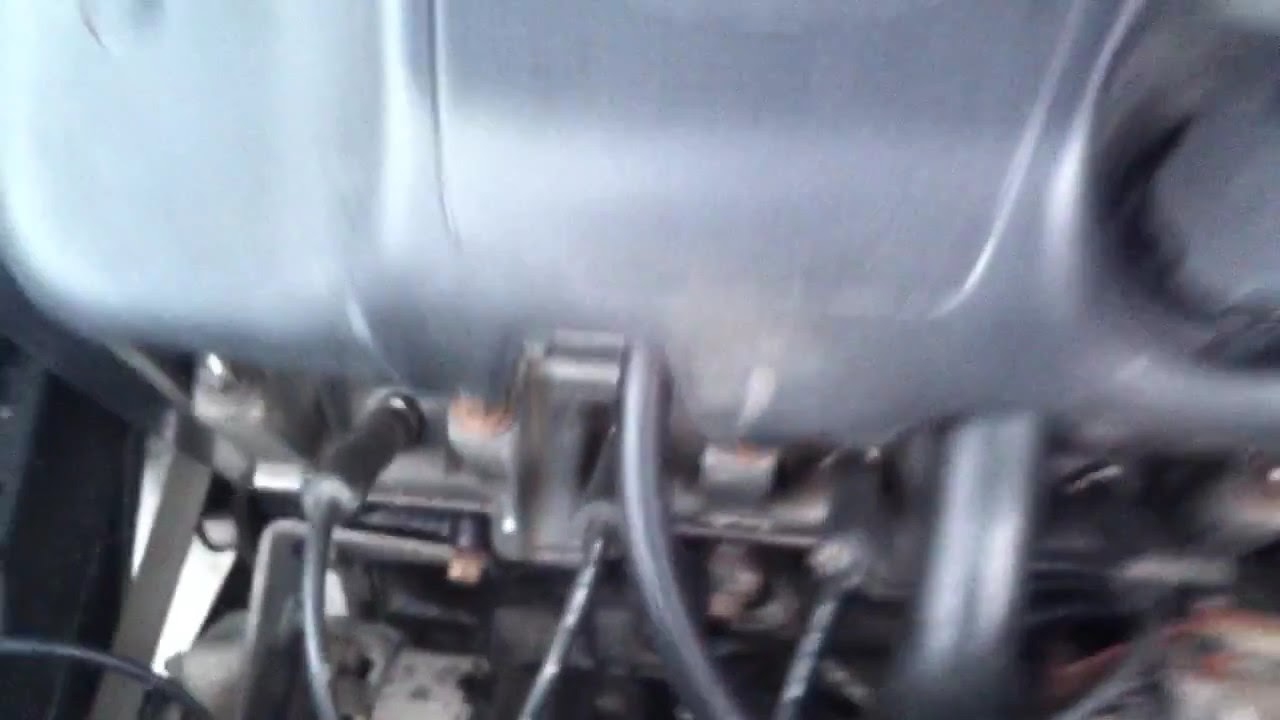This horizontal rectangular image is a close-up of a piece of machinery, heavily blurred due to camera motion. The top portion appears to be a solid metal surface or casing, reflecting light. The bottom section is more discernible, featuring a complex arrangement of wires and tubes in black and grey, with some red wiring visible. Various bolts, some slightly rusted, and multiple ports can be seen. On the right side, a screw-on cap and what might be a supporting leg are visible, suggesting this could be part of a tank or a similar structure. The background is dark, making it hard to determine the further details, but another leg might be present in the far right corner. Overall, the image gives the impression of the inner workings of a machine or vehicle, with a blurred metal shell housing various wirings and components.